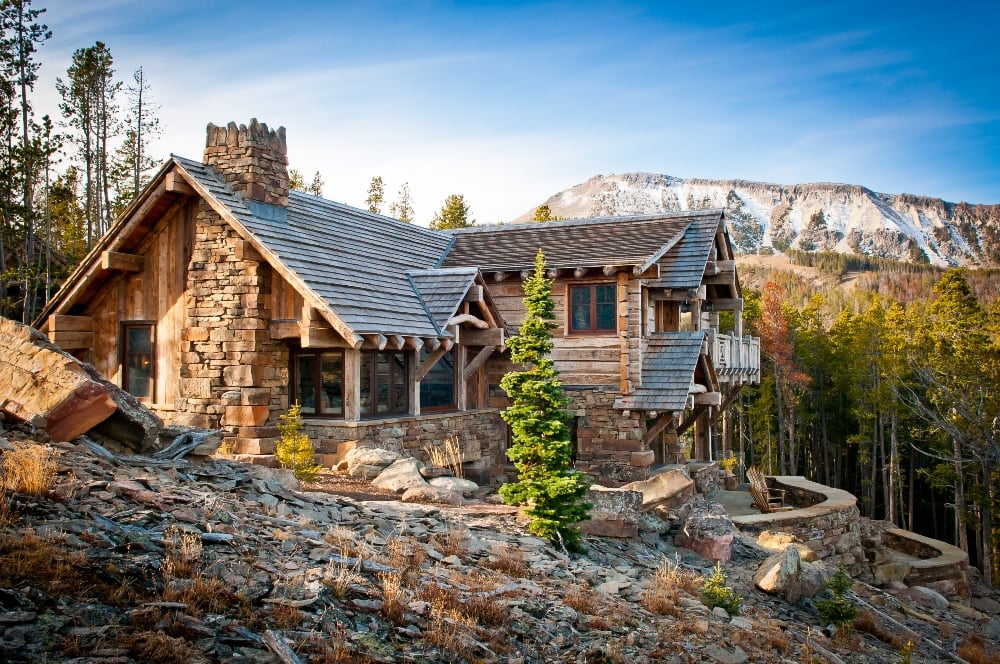In this detailed image, we see a rustic cabin situated on a slope in a mountainous region. The house is primarily constructed from old wood, with a stone base and a prominent stone chimney that extends from the bottom to the roof. The greyish-brown roof appears to be made of tin. The front of the house features wooden beams supporting the porch entryway, accompanied by several windows and a set of steps.

To the right of the house, we notice a small tree and a few chairs, suggesting a seating area. The terraced land around the cabin includes bare ground with stone terracing, indicative of the sloping terrain. The house's structure includes a wing with a slatted roof that covers a small deck enclosed with a wooden railing.

This dwelling appears to be a small, multi-roomed residence without provisions for parking. Surrounding the cabin are trees on both the left and right sides, with additional trees and mountains visible in the distant horizon. The scene is set under a blue sky with a few clouds, and the low sun casts a serene light across the landscape, emphasizing the rural and secluded nature of the setting.